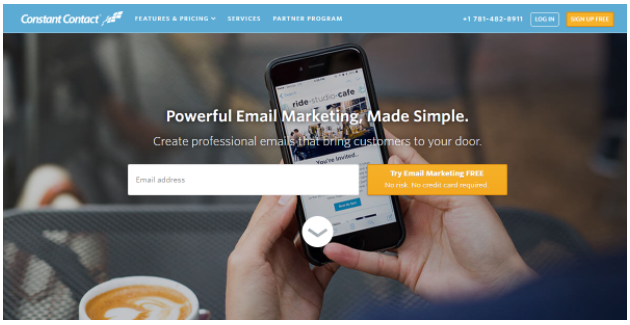The image showcased is from Constant Contact's website. At the very top of the page, a blue banner spans across the width, featuring white text. Notably, on the far right side of this banner is an orange rectangle button with the words "Sign Up Free." The name "Constant Contact" is prominently displayed alongside a small logo to its right. The banner includes options labeled "Features," "Pricing," "Services," and "Partner Program," as well as a visible phone number. Additionally, there is a white-lettered rectangle box that reads "Login."

Below the banner, an image features a person's hands holding a cell phone, angled slightly to the left. Superimposed on this image in bold white text are the words "Powerful Email Marketing made simple." Directly underneath, in non-bolded white text, it states, "Create professional emails that bring customers to your door."

Positioned below this text is a white rectangle input box with light gray lettering that says "Email Address," indicating where users can enter their email. To the right of this box, another horizontal rectangle, colored orange with white text, reads "Try Email Marketing Free. Risk free, no credit card required."

Centrally located on the page is a downward-facing gray arrow encased in a white circle. The background features a steel grated outdoor table. On the table, there is a caramel-colored coffee topped with cream, designed into two hearts or a flower and stem. The rest of the background is artistically blurred.